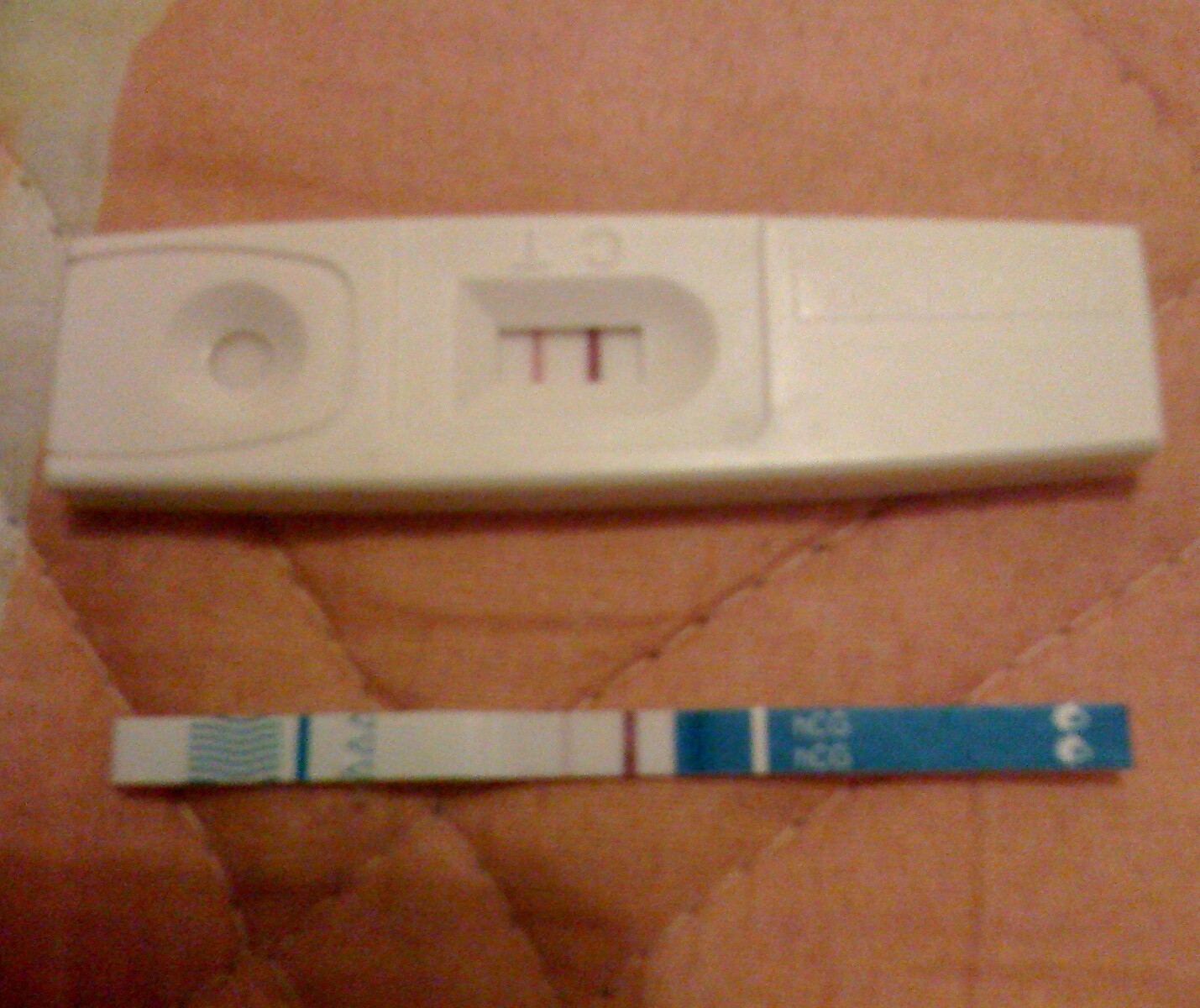This image showcases a COVID-19 test kit prominently displayed. At the top of the image is the actual testing card, which is made of white plastic and is rectangular in shape. In its current orientation, the card appears upside down. In the middle of the card, two small vertical lines are visible: the right line is a dark purple, while the left line is a light purple. Above these lines are the letters "C" and "T" respectively, where the "C" is located above the dark purple line and the "T" above the light purple line. In front of the testing card is a long test strip. The right part of this strip is dark blue, and the left part is white, adorned with blue curves and lines. This detailed arrangement highlights the components and results of the COVID-19 test kit.